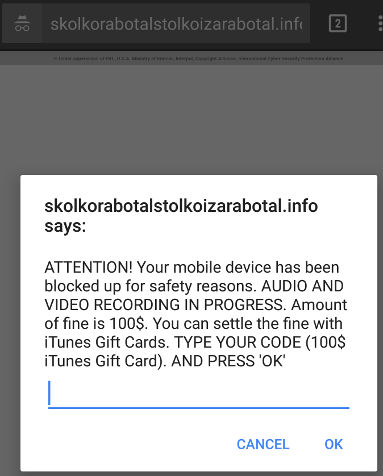This image shows a web browser on a mobile device displaying a suspicious website, "skolkoizabotal.info." At the top, the website address is visible in the browser's address bar. The screen features a pop-up notification warning the user that their mobile device has been blocked for safety reasons. The message claims that audio and video recording are in progress and instructs the user to pay a $100 fine using iTunes gift cards by entering the code and pressing OK. This is a clear example of a malware scam attempting to scare the user into making a fraudulent payment to unlock their device.